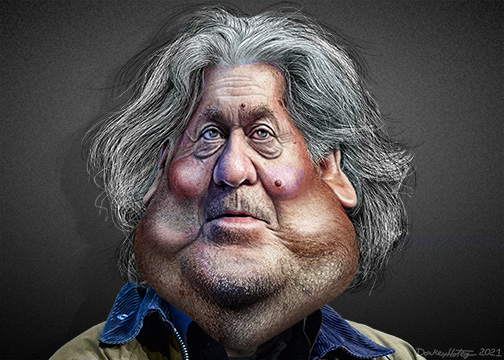The image is a caricature of a man with a distinctive, exaggerated face. His small forehead contrasts sharply with his very large jowls and chin, creating an almost triangular shape as his face widens dramatically from top to bottom. He has wiry, chin-length hair that is a mix of white, gray, and black, parted down the middle. His blue eyes are set above ruddy cheeks, and a mole is visible on his left cheek. The man appears unshaven, with stubble in the mustache and beard area.

He is dressed in a blue collar shirt beneath a beige jacket. The background of the image is a gradient of gray, lighter near his face and becoming darker toward the corners. There is a grainy texture to the background. In the bottom right corner of the image, the artist's signature is visible.

This caricature seems to be based on a modified or stylized photograph, perhaps altered using software like Adobe Photoshop to enhance the exaggerated features, particularly the enormous cheeks and chin.